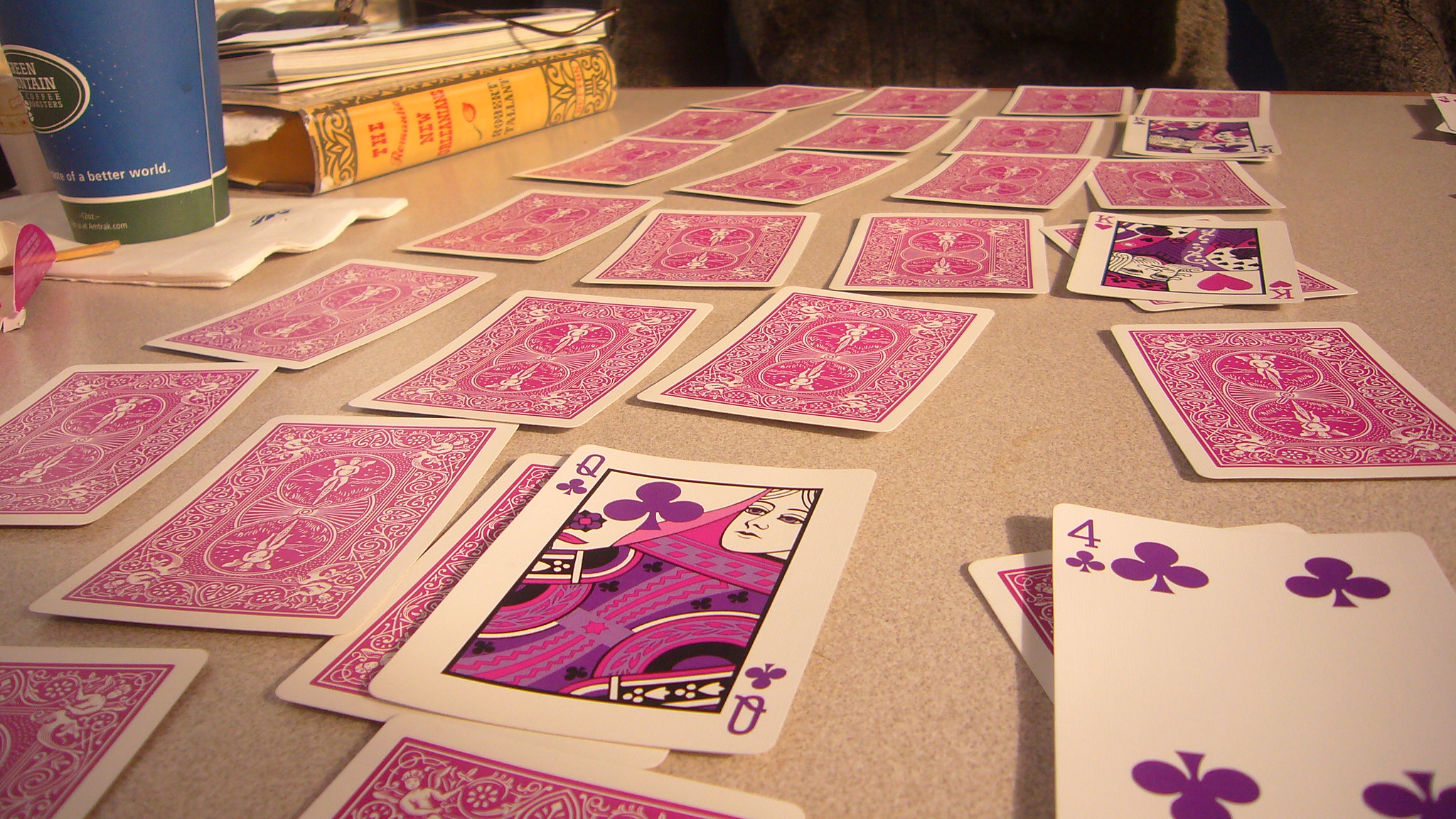The photograph depicts a light brown, textured tabletop captured from an extreme frontal angle, providing a flat point of view just above the table's edge. Arranged in an orderly manner, four rows of six playing cards each stretch away from the photographer. Notably, the playing cards appear faded, with an unusual pinkish hue, possibly due to significant wear or improper color correction in the photo. Among the visible cards are a queen of clubs, four of clubs, and king of clubs, interestingly all tinted red.

In the background to the left, a yellow-bound book lies horizontally next to another open book with its pages exposed. Atop these books rests a pair of glasses. A blue paper cup with a green bottom stripe and partially legible text reading "something mountain, something better world" sits alongside the books, hinting at a casual, possibly contemplative setting.